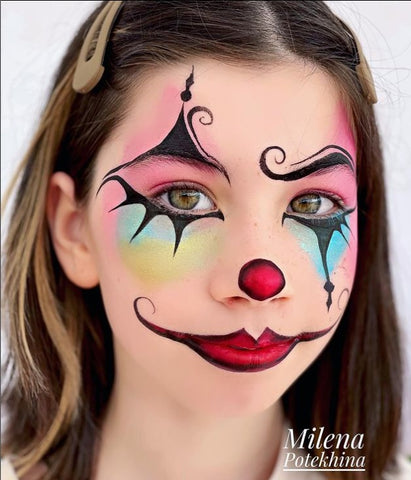The image features a close-up shot of a girl with shimmering green eyes and shoulder-length brown hair, held back by two brown hair clips on either side of her head. She is adorned in striking clown makeup: a big red circle with a black outline graces her nose, while her lips are painted a vivid red, similarly outlined in black, extending into an exaggerated, wide smile that curls outward. Her eyes are framed with a dramatic pink base above, and a blend of blue and yellow shades below, complemented by a black outline. Notable black, spiky lines extend downward from both eyes, as well as above her right eye, giving a bold, theatrical touch. Her eyebrows are brown, with the left one featuring a unique black triangular shape and a black curve at its start. This detailed and colorful makeup highlights the meticulous artistry, transforming her expression into one of whimsical enchantment.